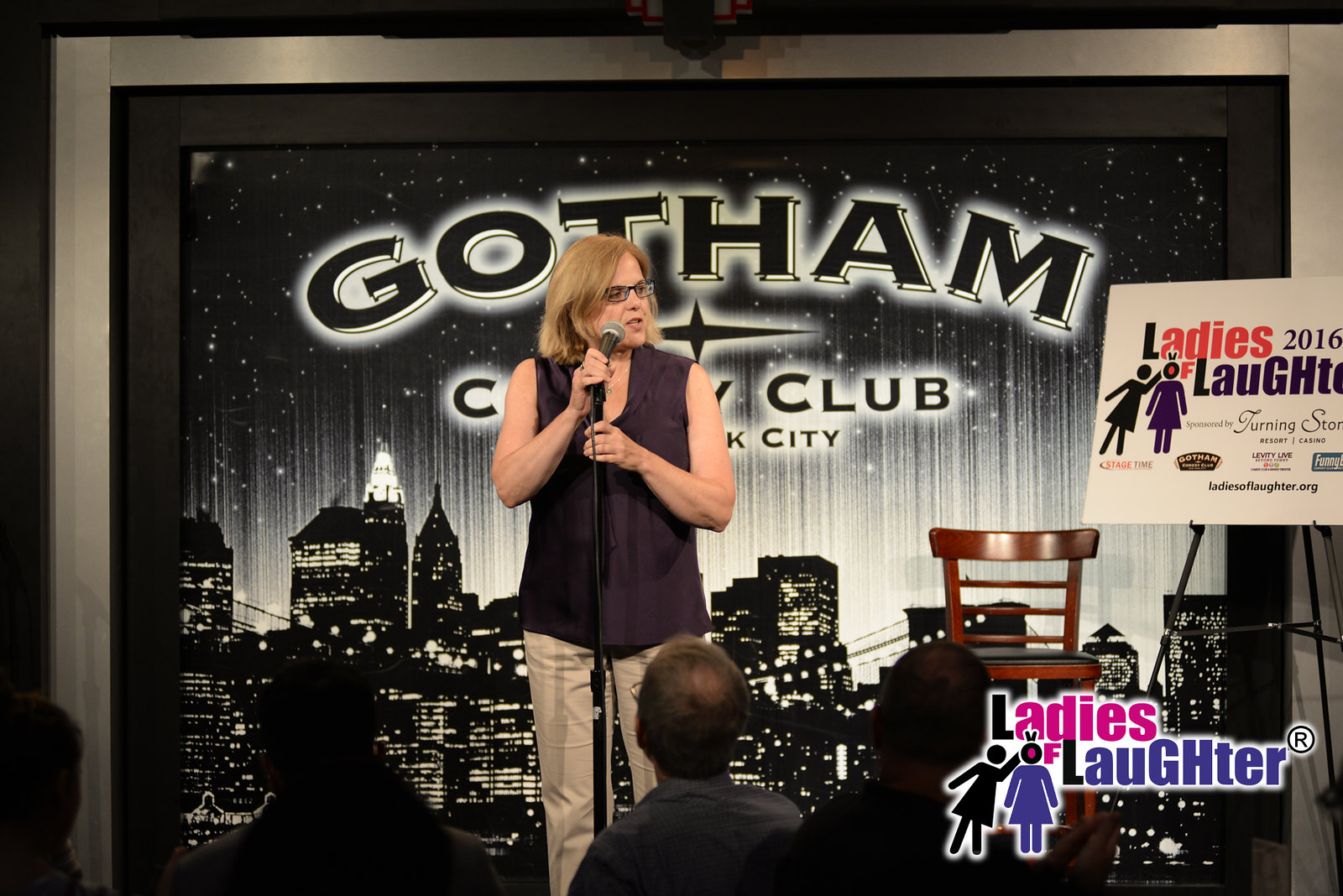The photograph captures a woman standing on a small stage, addressing an audience through a microphone on a black stand. She's wearing a black sleeveless top, khaki pants, and black-framed glasses. To her right, a wooden high chair with a black cushion is visible. The stage is framed by a small metal structure that encompasses an inner black frame, against a painted backdrop. The bottom half of the backdrop portrays a night-time cityscape with illuminated buildings and a bridge in the foreground, while the upper part features a night sky dotted with white stars. In bold black text with a white border, the words "Gotham City Club" are partly visible, partially obscured by the woman. Additionally, a panel on the lower right corner of the stage reads "Ladies of Laughter 2016," with a logo also saying "Ladies of Laughter." The composition suggests the image was taken from a raised vantage point at the back of the audience, showing the heads of seated viewers at the bottom of the frame.